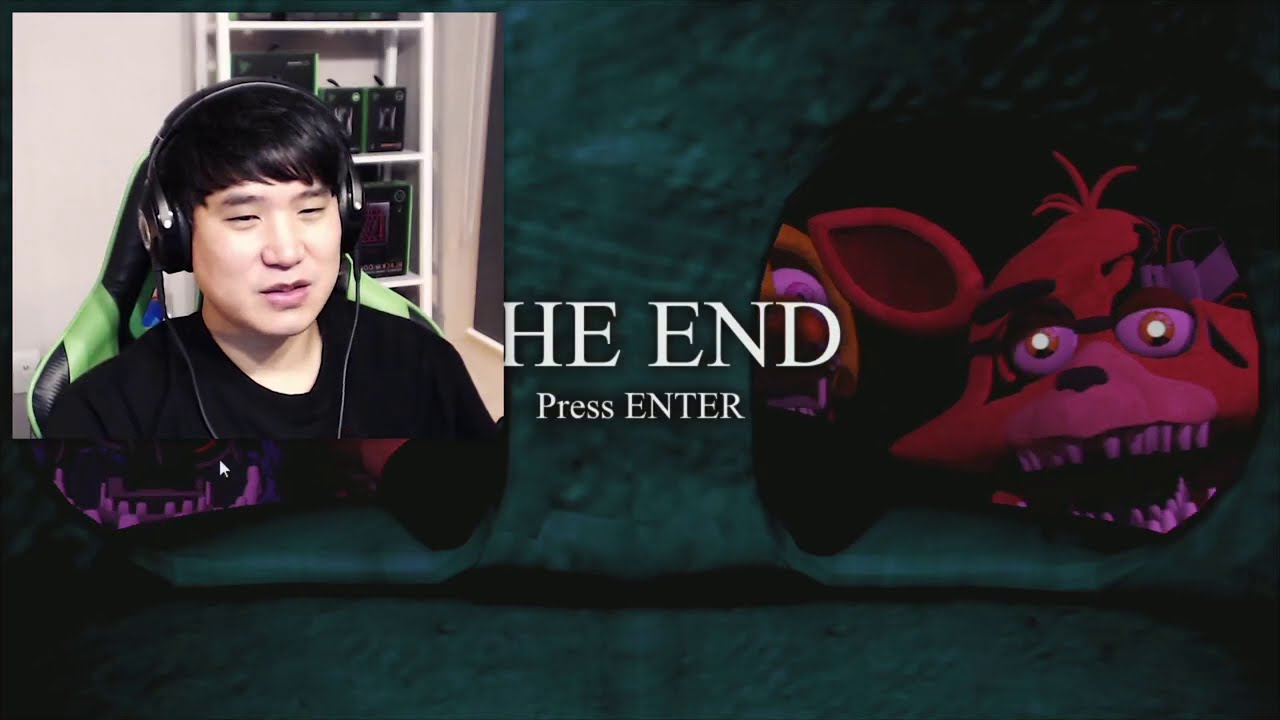The image is a still from a video game, likely Five Nights at Freddy's, showing a streaming setup. In the upper left corner, occupying about a third of the screen, there is an overlay of an Asian male streamer. He has black hair, is wearing a black t-shirt and headphones, and is seated in a green and black gaming chair. Behind him, there is a white shelf with black boxes that have green borders. The background of his room is beige. The main game screen displays the words "THE END" with "press enter" beneath it, imposed over a dark, greenish-gray stone-like texture. To the right, a creepy, animatronic red bear with glowing eyes ominously stands with its mouth open. The streamer appears disappointed or disgusted, perhaps due to losing the game.